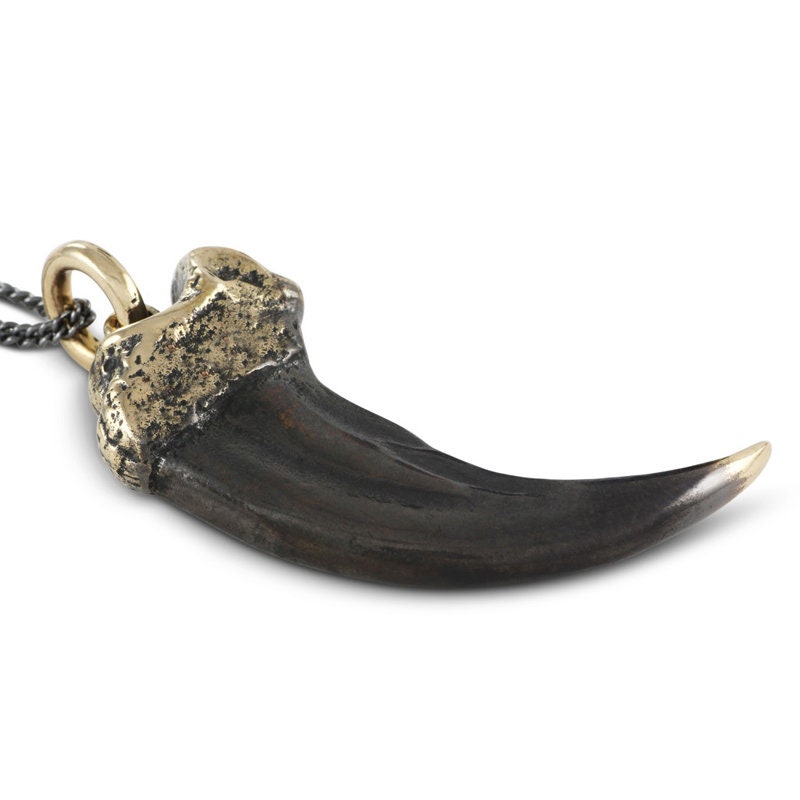The image features a close-up of a striking piece of jewelry—a pendant made from a curved animal tooth, perhaps from a shark or similar creature, displayed on a white background. The tooth is a deep, almost black color with a white to ivory tip, giving it a dramatic gradient. The tooth's root is encased in gold, resembling a dipped effect that leaves speckles of the original tooth color visible through the gold. A golden ring at the top of the tooth attaches it to a silver chain, adding a touch of elegance. The chain wraps around the gold hook, which is positioned on the left side of the image, enhancing the jewelry's intricate details in a manner suitable for a catalog or online store display.